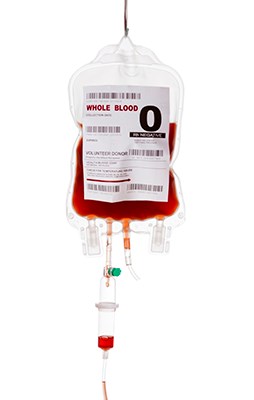The photograph shows a clear IV bag filled with a bright red liquid, labeled as "Whole Blood" with a prominent black letter "O" and the designation "volunteer donor." The bag is approximately three-quarters full. It hangs from a silver hook attached to its top center, which is fixed to a pole against a white background. The white label on the bag features several barcodes, including one at the top and four more scattered across the middle and bottom. Various ports are visible at the bottom of the bag; one connects to an IV line through which blood is seen dripping into a control area, and you can glimpse a small section of the tubing below that containing blood. One of the ports also appears to have a green plug and a syringe attached. The detailed setup indicates a meticulous arrangement for blood transfusion.